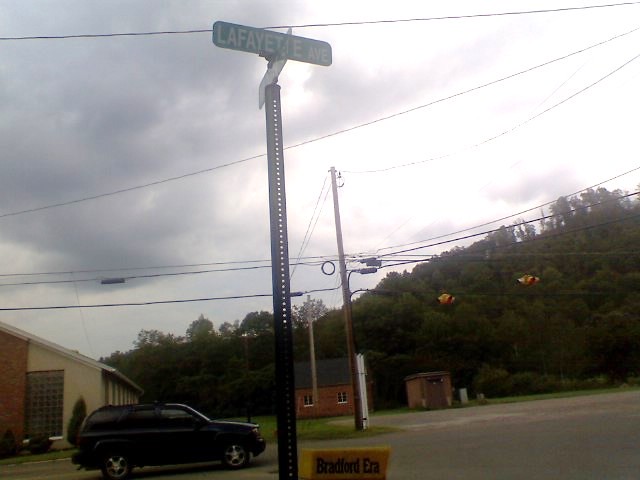The image captures a detailed street view set outdoors beneath a complex sky that is both blue and gray, filled with puffy white clouds and some darker areas, particularly in the upper left-hand corner where the clouds appear more foreboding. Sunlight filters through some of these clouds, giving the sky a dynamic appearance. Below the sky, a diverse tree line extends across the image, with varying heights and densities, some trees appearing lush and full, while others have sparse foliage.

Prominently featured in the foreground is a black SUV traveling along a road. Overhead, power lines stretch across the scene, intersecting the view with their geometric simplicity. Traffic lights with yellow casings and a green street sign indicating "Lafayette Ave" can be seen, providing context to the location. Another street sign is partially visible but the street name is not discernible.

Buildings line the street, including a light brown structure with a distinctive red brick section and a large window on its right side, situated in the left background of the image. A smaller, tannish-brown storage building with a dark brown door is also visible. In the distance, another brick building with a black roof can be seen near the center of the image, adding to the urban setting. Additionally, a yellow sign with black text that reads "Bradford Era" is visible on the right side of the image.